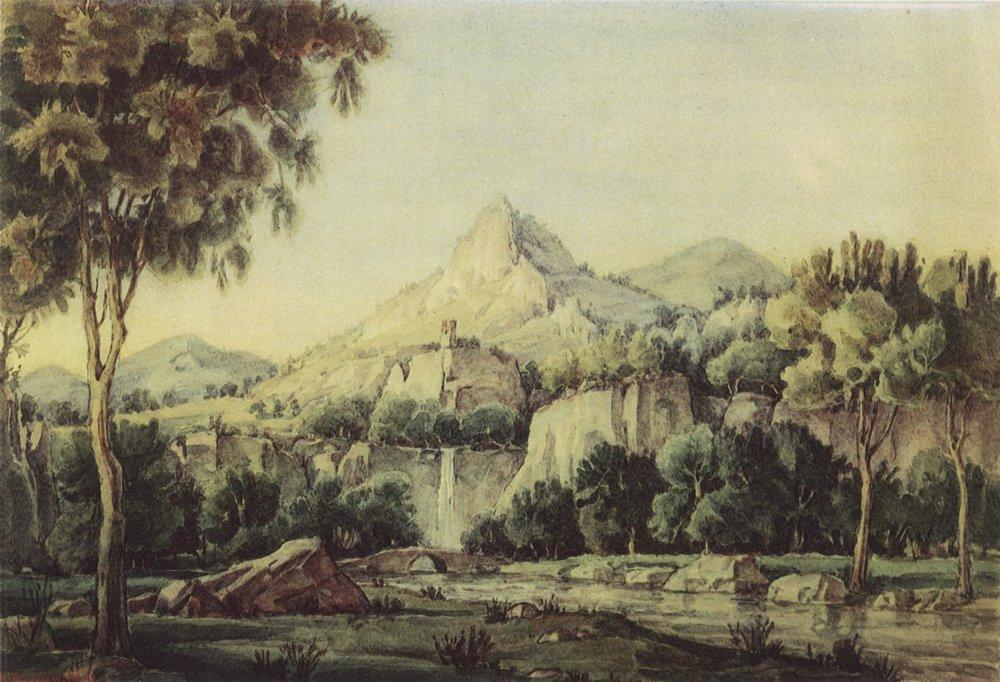The painting portrays a serene and sedate outdoor landscape, characterized by subdued, washed-out colors. Dominated by mountains in the background, the scene features verdant hues ranging from soft greens to darker shades that define various elements of the composition. In the foreground on the left, a single large green tree stands near a cluster of dark brown rocks. There are scattered small rocks and brush bordering a stream that flows from the lower right-hand corner towards the center, approximately 20-25 feet wide. A small stone footbridge arches over the river, which is flanked by grassy shorelines and lined with additional rocks.

On the right side of the painting, tall green trees, standing roughly 25-30 feet high, frame the landscape. At the base of the mountains, a waterfall cascades gracefully down the rocky slopes, adding a dynamic element to the tranquil scene. The sky above is populated with light blue and white clouds, and tinges of a faded dual green color, contributing to the overall calm ambiance. Additionally, the painting subtly incorporates a touch of architectural interest, with a distant, slightly indistinct castle or tower perched amidst the mountainous terrain, further enriching the scenic vista.